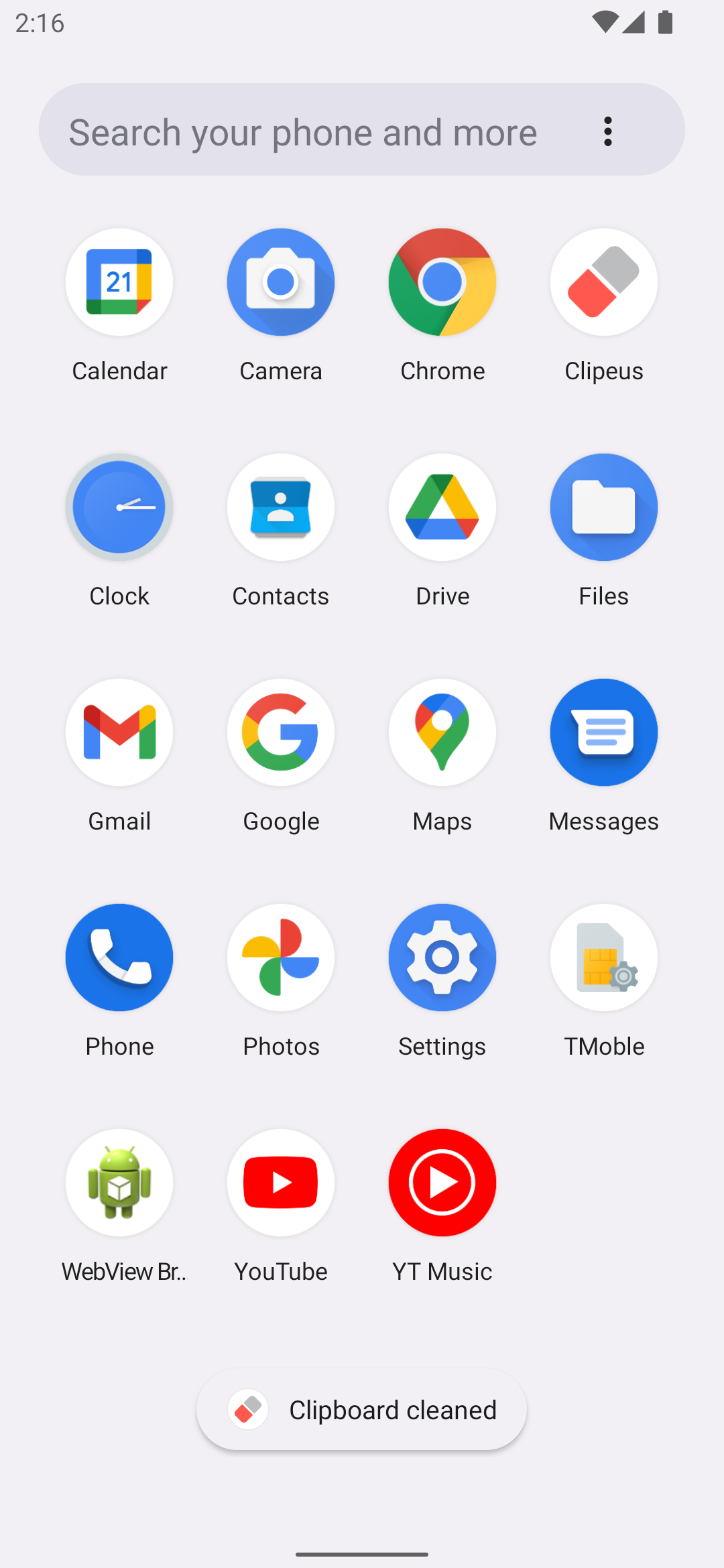The image displays a search interface on a mobile phone, featuring a search bar at the top that allows users to search their device and beyond. To the right of the search bar, there is an ellipsis (three dots), indicating additional options when selected. Below the search bar, a list of Google-related applications is presented in a vertical format, each accompanied by its respective, recognizable icon. The icons are visually consistent with Google’s color scheme and design standards, ensuring immediate recognition.

The listed applications include:
1. **Calendar** - Icon: A square with a calendar page design.
2. **Camera** - Icon: An outline of a camera.
3. **Chrome Browser** - Icon: A colorful circle reminiscent of a beach ball.
4. **Clock** - Icon: A clock face.
5. **Contacts** - Icon: A silhouette of a person.
6. **Drive** - Icon: A triangular motif in Google’s primary colors.
7. **Files** - Icon: A folder.
8. **Gmail** - Icon: An envelope bordered in Google red.
9. **Google** - Icon: A stylized 'G' in multiple colors.
10. **Maps** - Icon: A pin on a map.
11. **Messages** - Icon: A speech bubble.
12. **Phone** - Icon: A traditional telephone receiver.
13. **Photos** - Icon: A multi-colored pinwheel flower.
14. **Settings** - Icon: A gear.
15. **T-Mobile** - Icon: A stylized 'T'.
16. **Webview Browser** - Icon: A globe.
17. **YouTube** - Icon: A red rectangle with a white play button in the center.
18. **YouTube Music** - Icon: A play button inside a circle.

At the bottom of the list is a "Clear Clipboard" button, easily identifiable for maintaining organizational efficiency on the device. Each icon not only follows the conventional design synonymous with its service but also employs the familiar color palette associated with Google's branding, facilitating user navigation and recognition.